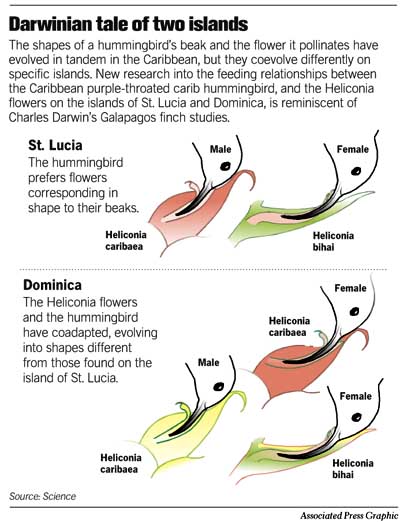The image, set against a white background with black text, is titled "Darwinian Tale of Two Islands" and contains illustrative panels detailing the co-evolution of the Caribbean purple-throated Carib hummingbird and Heliconia flowers on the islands of St. Lucia and Dominica. The central thesis, reminiscent of Charles Darwin's Galapagos Finch studies, explains how these birds' beaks and the flowers they pollinate have evolved in tandem, but with specific differences based on their islands.

The top portion of the image focuses on St. Lucia, where the male and female hummingbirds have beaks evolved to fit the shapes of the Heliconia caribea and Heliconia beehai flowers respectively. An illustration shows a male hummingbird with a straight beak sipping nectar from a pink Heliconia caribea flower and a female with a longer, curvier beak accessing nectar from a green Heliconia beehai flower.

A dotted line separates this from the Dominica section, where the Heliconia flowers and hummingbirds have co-adapted differently. The illustrations depict a male and two females with varying beak shapes, engaging with differently colored Heliconia flowers. The text notes that these evolutionary adaptations are distinct from those observed on St. Lucia, highlighting unique ecological dynamics. The image, credited to the Science Associated Press Graphic, serves as an educational insight into the adaptive relationships between these hummingbirds and their preferred flowers on both islands.